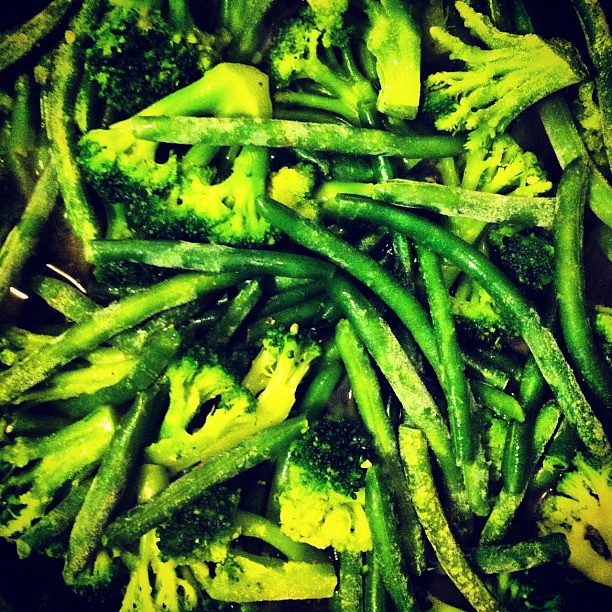This square-shaped photograph features a vibrant medley of fresh green beans and broccoli on a black background. The vegetables appear to be partially cooked, likely to an al dente consistency, showcasing their bright and natural green colors. However, the photo's hue appears to have been edited, with some parts of the broccoli stalks displaying an almost unnatural yellow tint. The mixed vegetables seem to be either cooking or resting on a surface, possibly a skillet or a plate, given the presence of a liquid underneath them. This liquid could be water, cooking oil, or even a sauce. The seasoning is evident with a white, powdery substance sprinkled over the vegetables, which might be Parmesan cheese, though the edited colors cast some doubt on the true appearance. The overall composition shows only the broccoli and green beans in a lush, green, and slightly yellow presentation against the stark black backdrop.